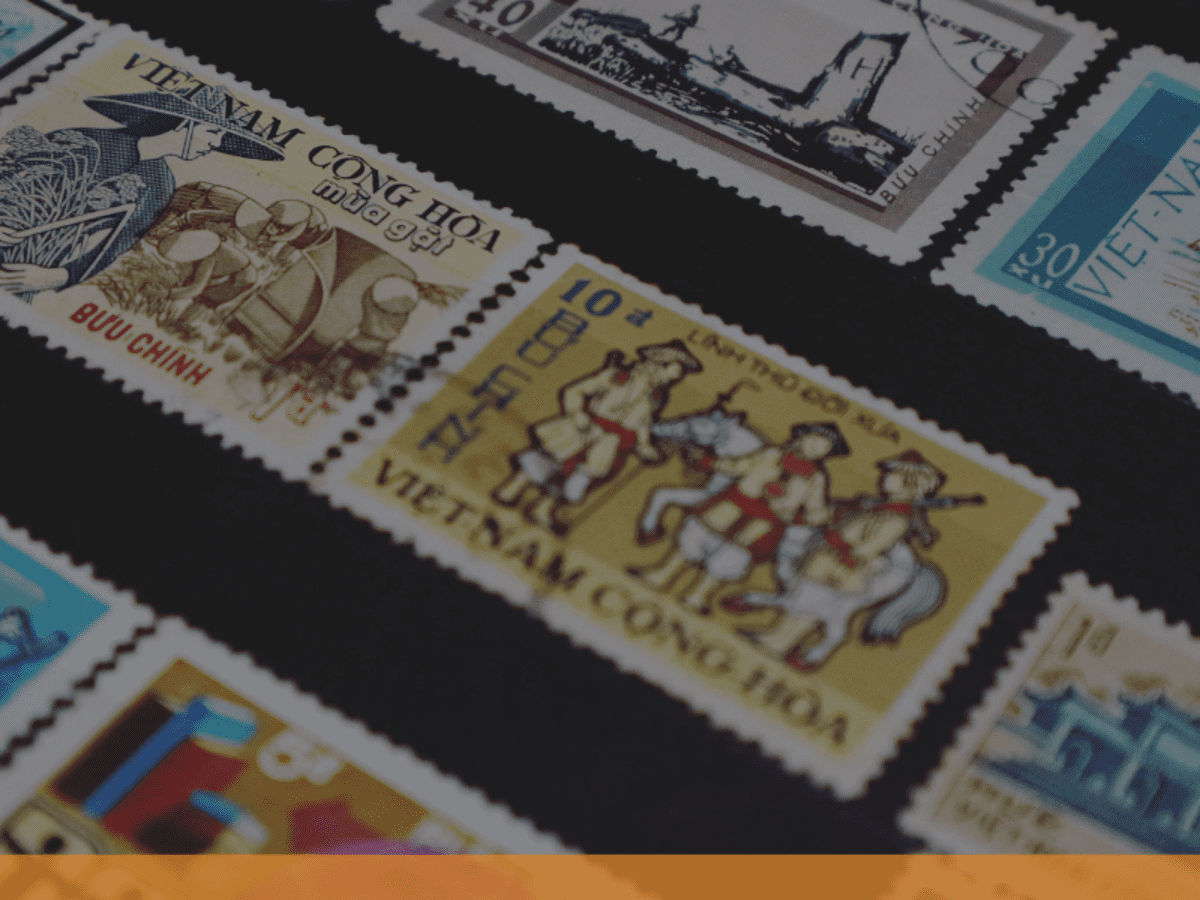This is a detailed, square, full-color photograph of a Vietnamese stamp collection, likely taken indoors. The image is arranged with the stamps positioned at an angle, descending from the top left to the bottom right, displayed against a black background. The photograph features three clear rows of stamps, with a prominent light orange border running horizontally along the bottom.

The collection showcases a variety of stamps, all rectangular with jagged edges. Two stamps in the middle row are particularly noteworthy. The first stamp on the left is primarily light yellow and features an Asian person wearing a traditional rice hat, depicted in blue. The text on this stamp reads "Vietnam Cong Hoa" at the top, "MUA GAT" in the middle, and "BUU CHINH" at the bottom in red. The image also illustrates people working in a rice field.

To the right of this stamp is another, more yellow in color, depicting three men in traditional dress, wearing conical hats, with one man appearing to have a gun slung over his shoulder. Behind them, there is a white horse. This stamp also reads "Vietnam Cong Hoa" at the bottom, with the number "10" situated at the top left in blue.

The overall presentation suggests these stamps are part of a meticulously organized and cherished collection, possibly housed in a collector's book.